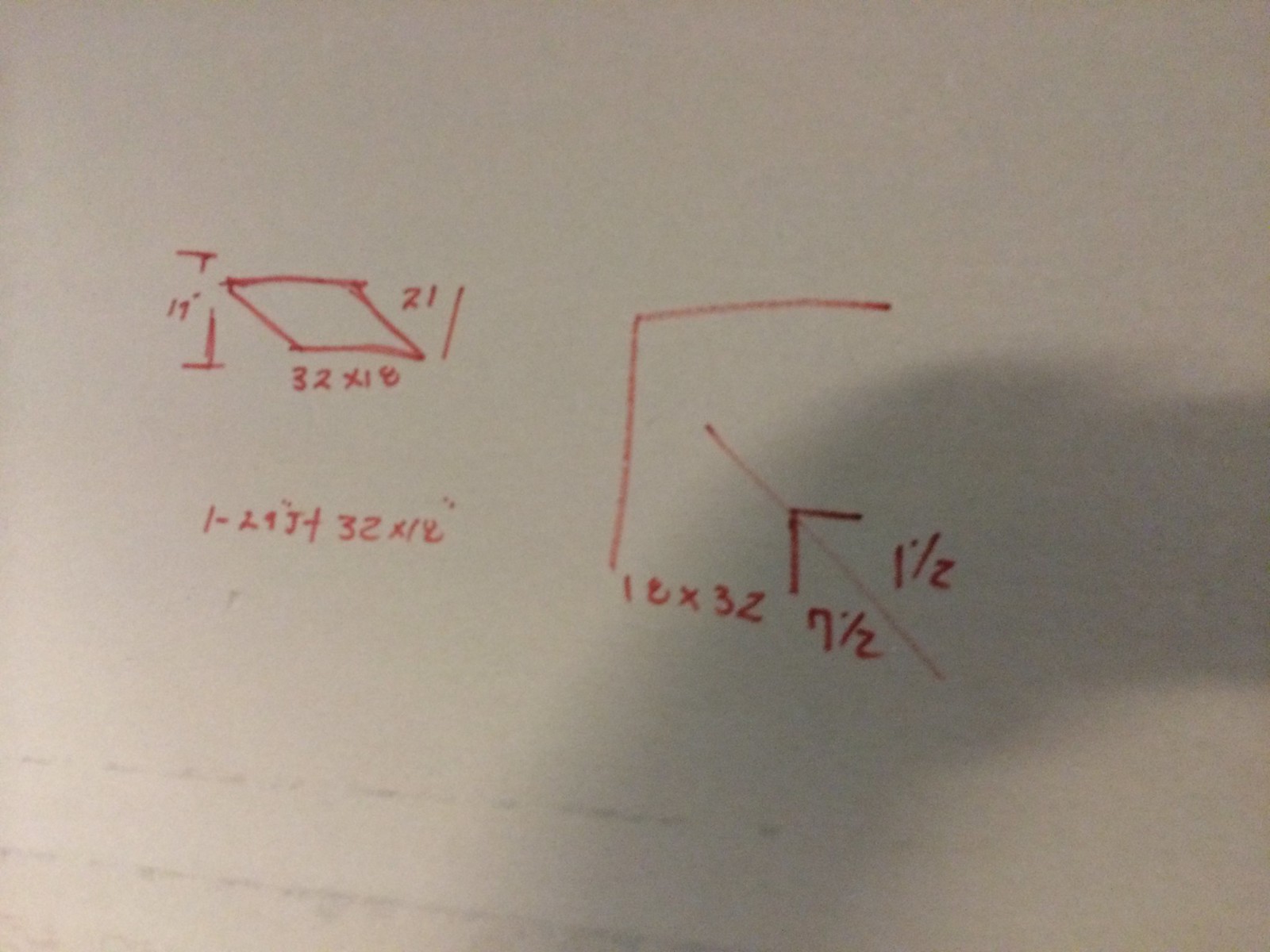A whiteboard (or piece of paper) is depicted with a detailed mathematical equation and figure drawn in red ink or red magic marker. The left side features a parallelogram with a base labeled "32 times 18" and a height possibly indicated by a vertical line labeled "21". On the right side, there are two right angles: a larger one and a smaller one, connected by a diagonal line forming an arrow shape. Below these angles, some notations include "18 times 32", "7 and a half", and "1 and a half", alongside some other complex mathematical expressions like "1 minus 29j plus 32 times 12". Additionally, there are indications of measurements, such as "19", which appears to denote a distance of 19 feet based on the accent mark.